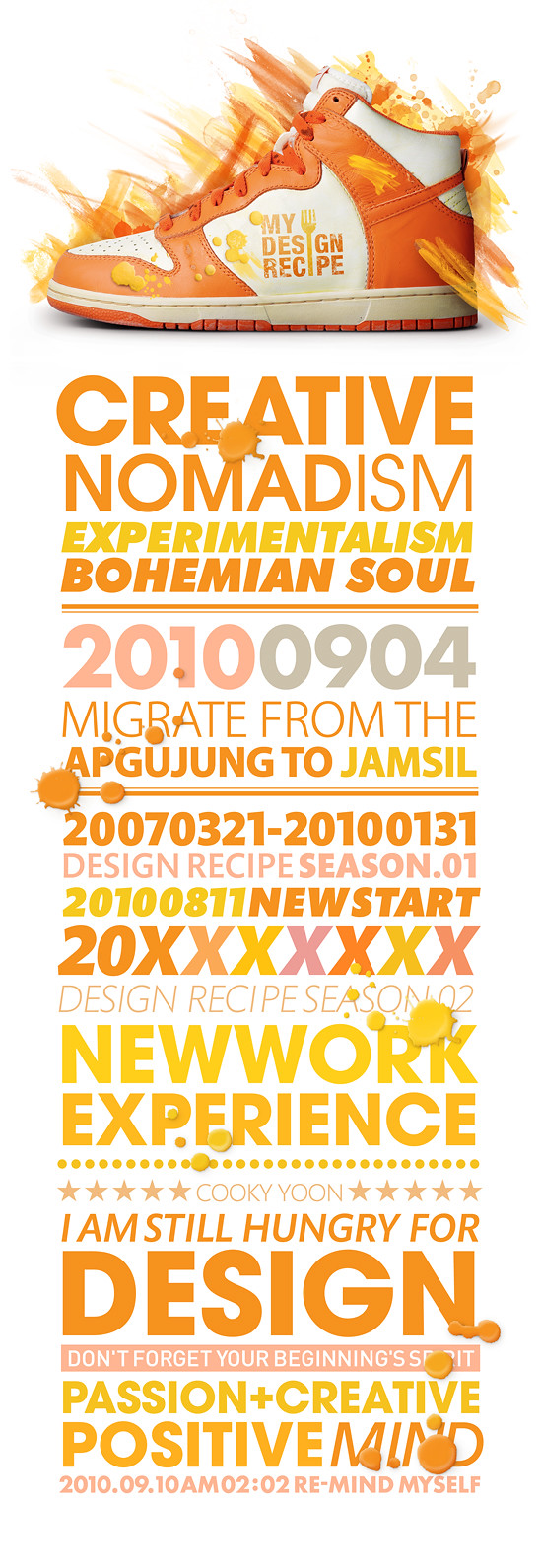The image appears to be an advertisement or promotional flyer, predominantly using bright orange and yellow hues in its text and design. It has a white background and features a digitally rendered side profile of an orange and white tennis shoe with a stylized, artistic approach. The shoe is positioned towards the left with its toe pointing leftward. Surrounding the shoe are vibrant orange paint splotches. At the top of the image, in orange text on the sneaker, it reads "My Design Recipe."

Below the shoe, a series of texts in various shades of orange, yellow, and some purple convey a creative and experimental theme. The main bold text states "Creative Nomadism, Experimentalism, Bohemian Soul." Further down, several date sequences, such as "2010-09-04" and "2007-03-21 to 2010-01-31," appear among other information. Phrases include "Migrate from Apgujeong to Jamsil," "Design Recipe Season 01," "New Start," and "Network Experience." The name "Cookie Yoon" is also mentioned along with motivational phrases like "I am still hungry for design," "Don't forget your beginnings," and "Passion plus creative positive mind."